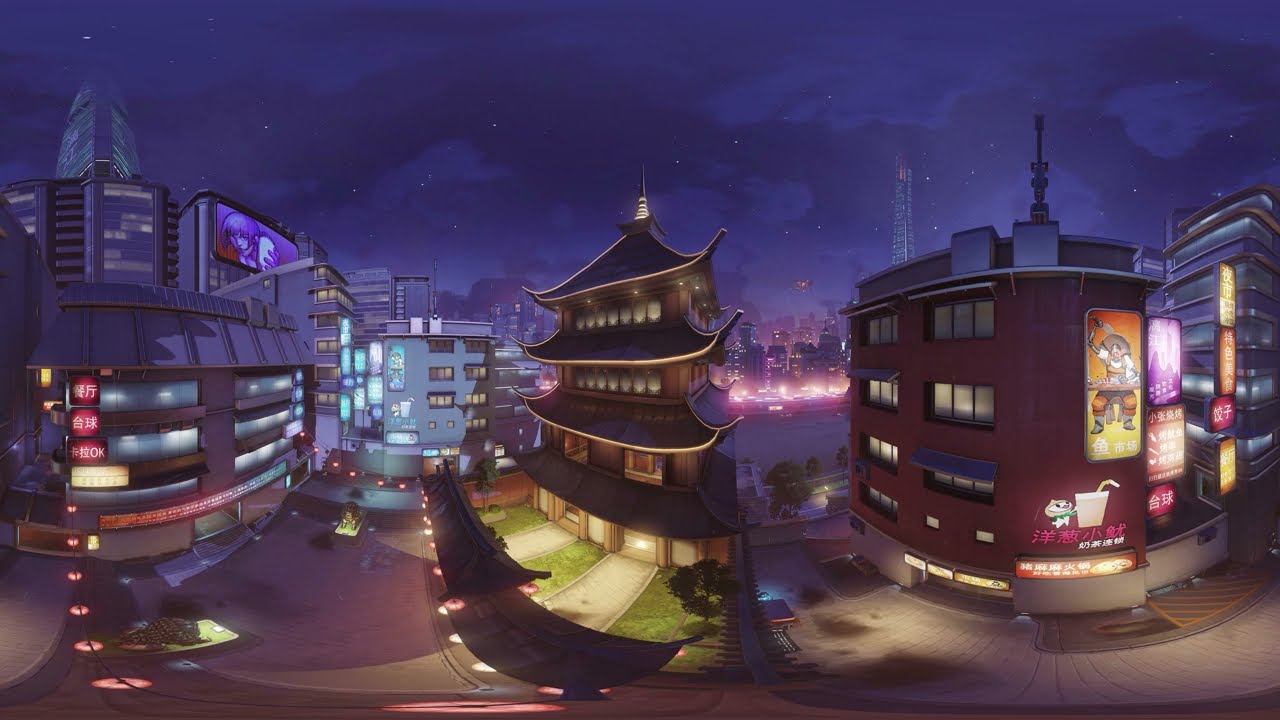The image is a digitally created, surreal nighttime scene of an Asian city, likely Chinese due to the numerous Chinese characters on neon signs and billboards adorning the buildings. The sky is a rich blend of blue and purple hues, dotted with scattered clouds and stars, reinforcing the nighttime setting. The city's architecture is eclectic, with buildings featuring both modern and traditional Chinese designs, including a prominent four-story structure resembling a traditional Chinese hut. The scene includes various advertising signs, many in vibrant colors such as red, purple, yellow, and orange, displaying animated characters, an anime girl, and other decorations. The foreground shows a fenced-in area and driveways suggesting possible residential use, while the background reveals towering skyscrapers illuminated by street-level lights. The cityscape exhibits no traffic or people, heightening its serene yet artificial ambiance. Small areas of greenery with grass and trees are also visible, interspersed among the urban structures.